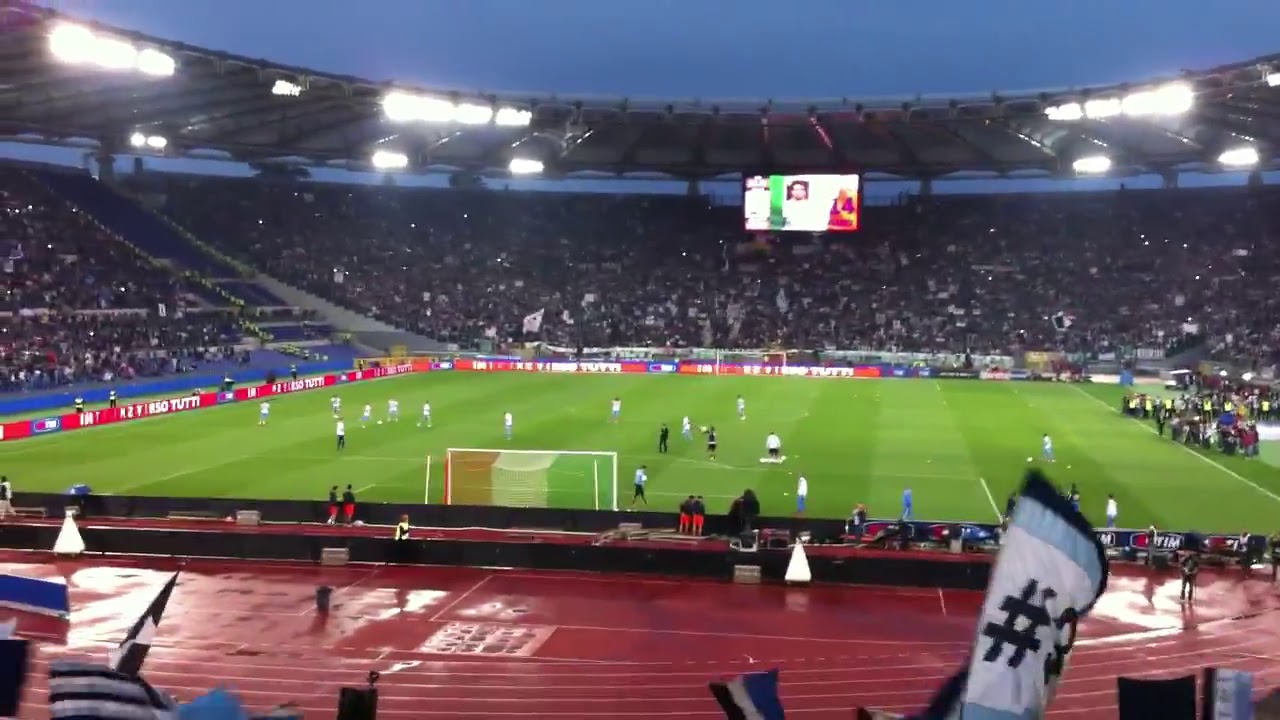The image captures a vibrant evening scene at a large, open soccer stadium. The sky above is darkening to a deep blue, hinting at the approaching nightfall, while powerful stadium lights illuminate the venue. The green soccer field, meticulously maintained with short grass, sits at the heart of the stadium, framed by a red running track that reflects the floodlights. 

Players wearing white and blue jerseys are competing on the field, with goalies positioned in front of vividly colored nets that feature green, white, and red hues. Some individuals in black uniforms are visible on the sidelines, possibly officials or team members. Surrounding the field is a red barrier adorned with dynamic LED advertisements. 

The stadium is filled with an immense crowd, occupying nearly every seat, and many are seen standing, cheering, and waving flags. Above the packed stands is a gray roof adorned with additional large lights, ensuring the entire arena is well-lit. A large LED screen further engages the audience by displaying relevant game information. The image captures the excitement and energy of a live sporting event in a grand, multi-purpose stadium.